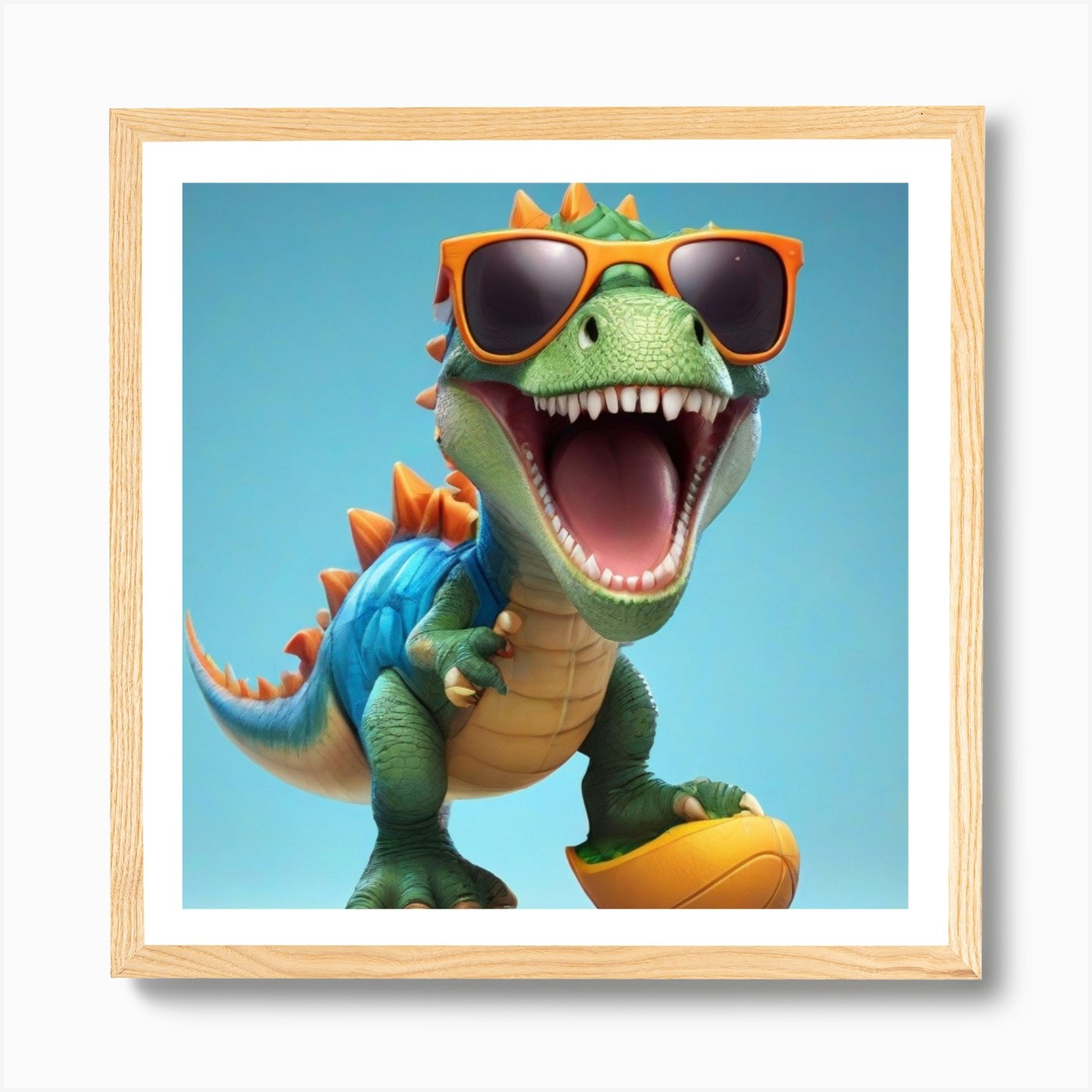The image depicts a colorful drawing framed in unfinished wood, set against a plain white background. In the picture, there is a whimsical dinosaur character predominantly colored green with a striking blue tail and back. The dinosaur is adorned with golden spikes that run along its entire back, adding a touch of fierceness to its appearance. It sports a pair of bright yellow shoes that resemble water skis and wears yellow sunglasses with black frames, effectively concealing its eyes. The dinosaur's wide, upward-curved mouth reveals a set of sharp white teeth, contributing to its playful, smiling demeanor. The background surrounding the dinosaur is a solid blue, making the character stand out vividly.